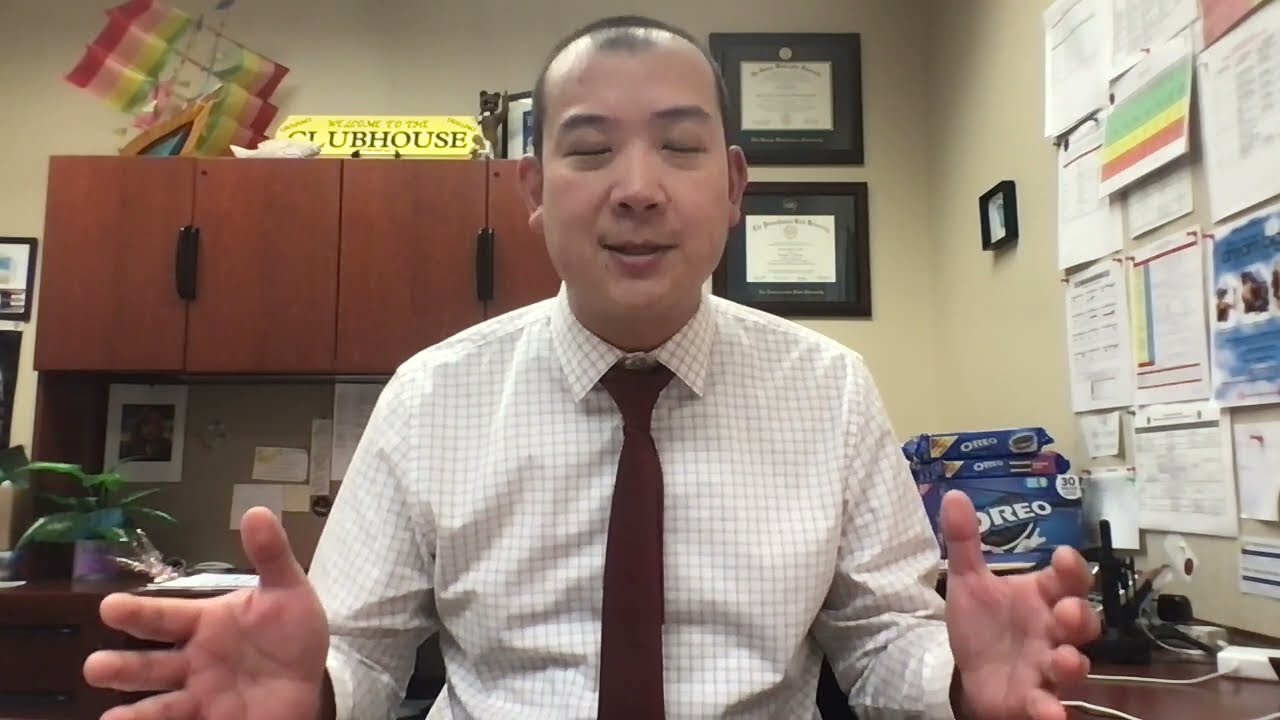In this detailed image, we see an Asian man, likely middle-aged, positioned centrally and appearing to prepare for speech despite having his eyes closed. He sports thin, balding black hair, black eyebrows, and has no facial hair. His attire consists of a white button-down shirt with a grid-like pattern of dark horizontal and vertical lines, complemented by a slim, maroon tie. His hands are open with palms facing each other, suggesting an expressive gesture or imminent conversation.

The setting is an indoor office, marked by an array of personal and professional items. Behind the man, there are deep brown cupboards with black handles and a stack of Oreos. To one side, the office wall is adorned with various papers and red thumbtacks, alongside two framed diplomas that signify his academic achievements. A small green plant in a purple pot sits on a desk, also visible in the background, with its large green leaves adding a touch of color. The scene is filled with colors such as red, orange, yellow, green, brown, white, maroon, and blue, all contributing to the office's busy yet organized ambiance. A "Welcome to the Clubhouse" sign on the wall further personalizes the environment, indicating a warm, inviting workspace.